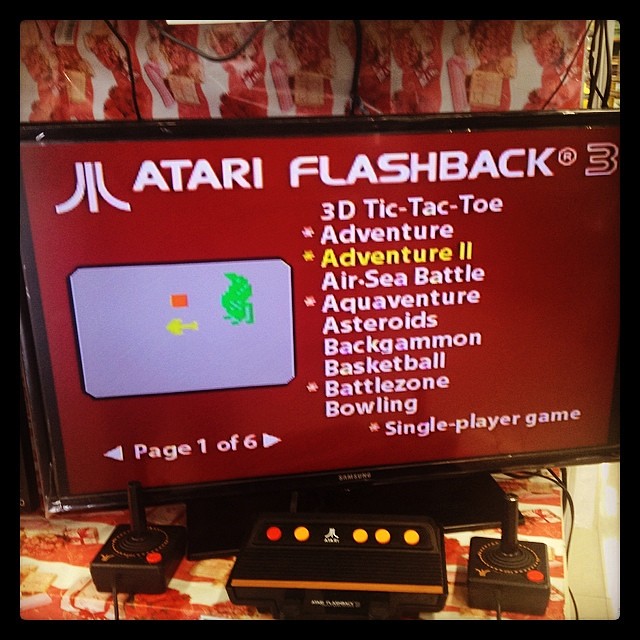The photograph features a flat-screen television displaying the menu of the Atari Flashback 3 game system. Below the television, the Atari console is visible alongside two joystick controllers featuring red fire buttons. The console itself has five buttons: a prominent red power button, and four other buttons likely for game selection. The classic Atari logo is positioned centrally on the unit. 

The television screen shows the title "Atari Flashback 3" with game titles listed beneath, including "3D Tic-Tac-Toe," "Adventure," "Adventure 2," "Air-Sea Battle," "Aquaventure," "Asteroids," "Backgammon," "Basketball," "Battlezone," and "Bowling." Some games are marked with asterisks to denote single-player options. This is the first of six pages in the game menu. The menu background features a deep red hue, adding a nostalgic touch to the display.